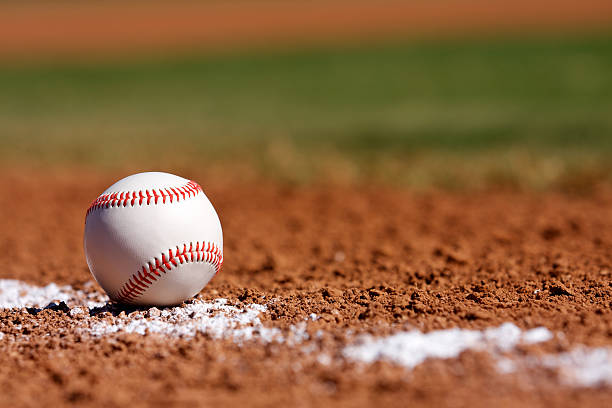This image captures a close-up view of an exceptionally clean, white baseball with red stitching, positioned on a chalk line amidst a baseball diamond's dirt surface. The baseball sits predominantly on the lower to middle left side of the frame, slightly shadowed on its left due to sunlight streaming in from the right. The white chalk line runs horizontally across the image, from left to right, though partially covered with dirt gravel. The background features a blurry mix of green grass and brown dirt, hinting at the field's boundary, with the green sandwiched between the blurred brown portions. The overall setting suggests the photo was taken in the evening, with warm sunlight enhancing the baseball's pristine appearance against the earthy tones of the diamond.